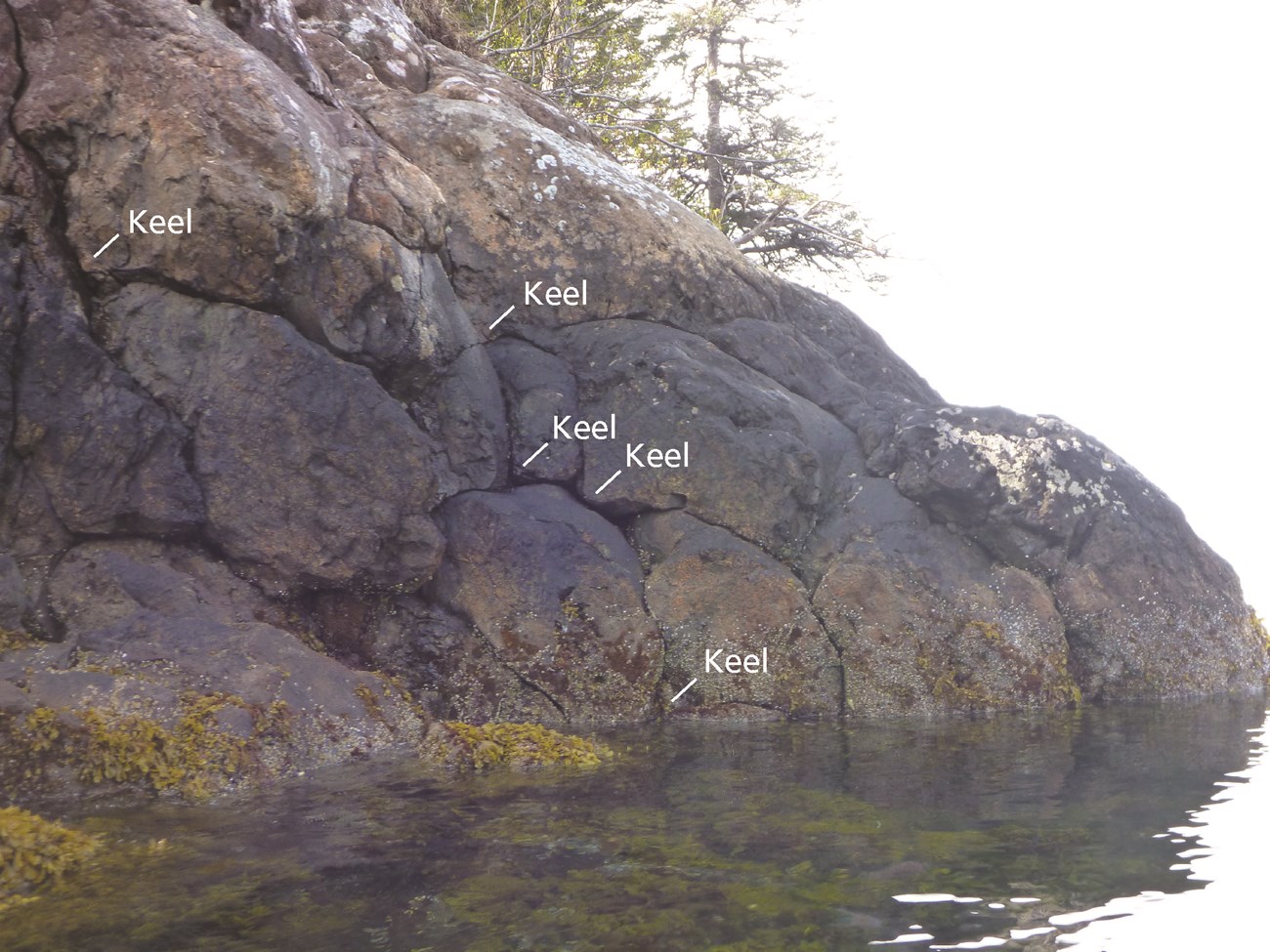In this outdoor daytime scene, a large rock formation dominates the lower half of the image, with calm water at its base. The rock, exhibiting a mix of light brown, dark brown, and gray tones, features several white labels marked "Kiel," with arrows pointing to cracks and divisions in the boulders. These labels appear five times, primarily clustered in the center of the formation. A spread of moss can be seen in the water near the rock, with some of the moss appearing yellowish-green. Extending from the left upper corner to the middle right of the picture, the rock formation is flanked by trees that line the background from left to right. The sky occupies the upper right corner of the image, forming a triangular patch of plain white, contributing to the serene atmosphere. The bright sunlight from the right illuminates the scene, casting reflections in the calm water below.